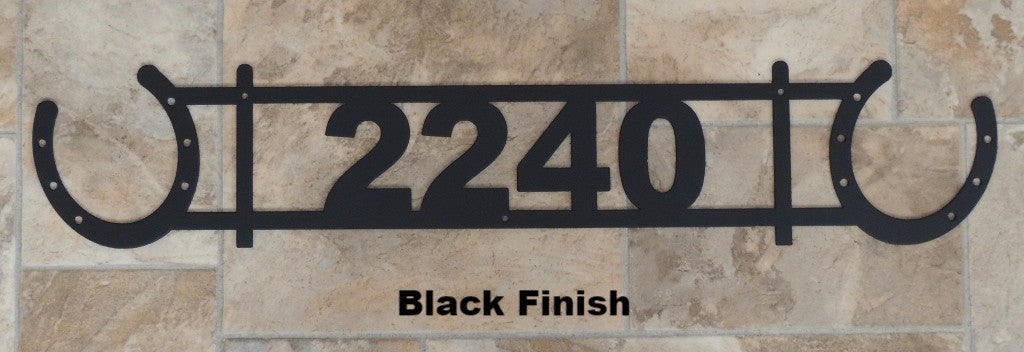This image is a professionally crafted address marker designed for exterior use. It prominently features the house number "2240" in a black finish, elegantly framed by two upward-angled horseshoes on either end, each pierced with six decorative holes. The marker, made of wrought iron, includes additional mounting holes for secure attachment. The background showcases a marbled beige, tan, and cream tile floor with clear gray grout, emphasizing the marker's sophisticated design. The overall composition of the photograph centers the marker against this visually appealing backdrop, illustrating its potential placement on a wall.